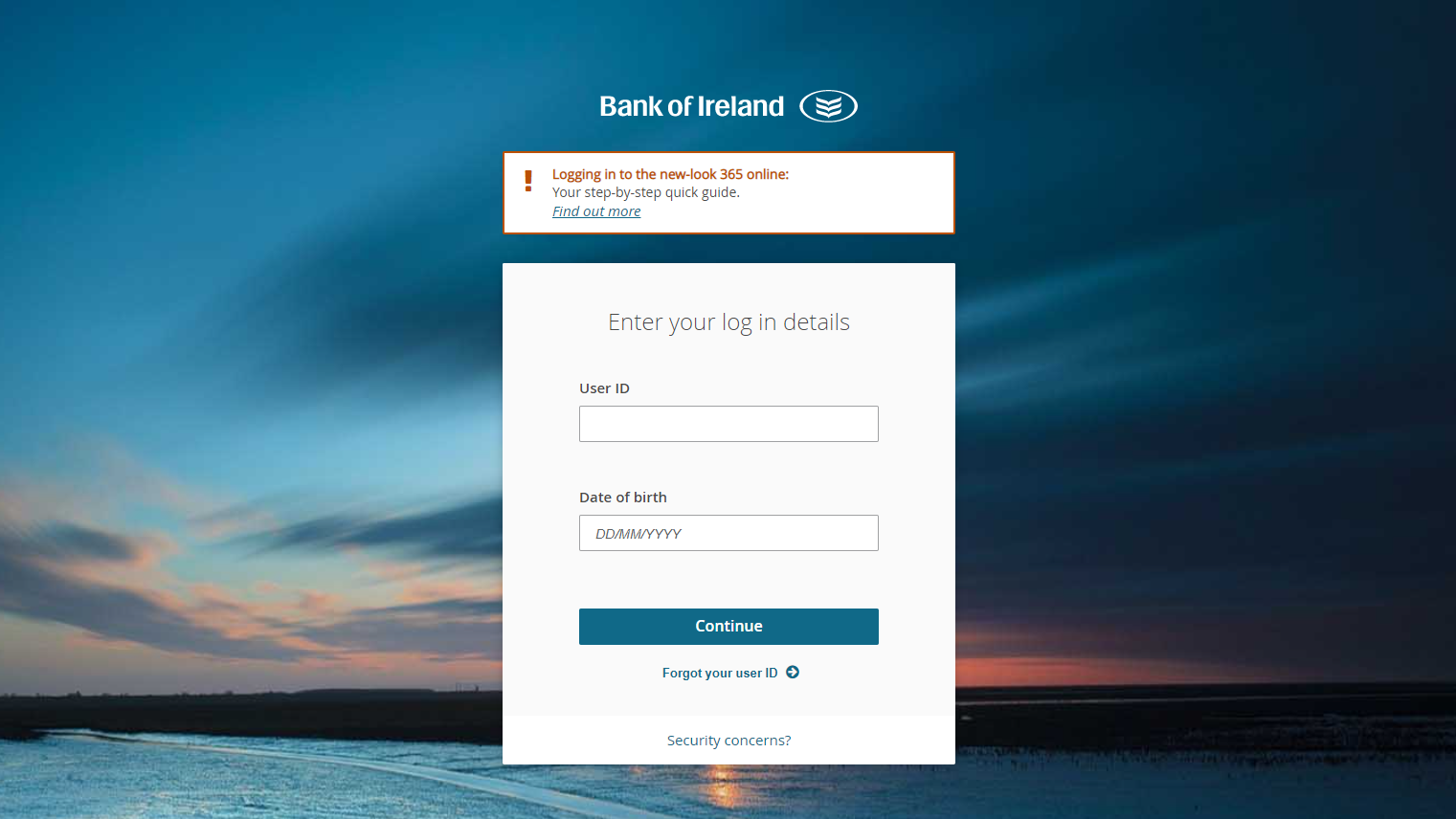This image depicts a desktop screen featuring a login page, likely for an online banking platform. The background consists of a serene sunset or sunrise scene, with a gradient sky showcasing hues of blue, gray, pink, and orange, gradually blending together. Below the sky, the ocean is visible, displaying various shades of blue water illuminated by the sunlight.

In the foreground, the login interface prominently displays the branding of "Bank of Ireland," accompanied by a logo of three arrows arranged in a circular pattern. A red exclamation point icon within a red-outlined white box highlights an important notice, reading: "Logging into the new look 365 online, your step-by-step quick guide." A hyperlink is provided for users to find out more.

Below this notice, the login area consists of a white box prompting users to enter their credentials. The first input field requests a "User ID," followed by a "Date of Birth" field using the format date/month/year. A blue "Continue" button is situated below these fields. Additional options include a clickable "Forget your User ID?" link with an arrow pointing to the right, and a "Security concerns" link, offering quick access to help for users with login issues.

The overall scene suggests that someone is attempting to log into their Bank of Ireland online account amidst a visually appealing and tranquil backdrop.